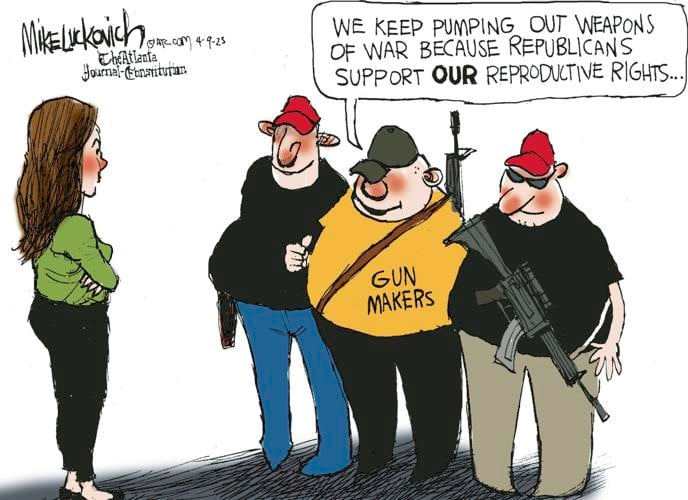In a highly detailed cartoon illustration by Mike Lukovich from the Atlanta Journal-Constitution, dated 4/9/23, a scene unfolds on a gray street against a white background. The focal point is a woman with long brown hair, wearing a bright green long-sleeved shirt, black pants, and black flats. She stands with her arms crossed, staring indignantly at three men, who are depicted as overweight and somewhat dimwitted. These men, all gun makers, hold rifles and are dressed in hats, with two in black shirts and one in a yellow shirt that bears the text "Gun Makers." They collectively speak from a speech bubble that reads, "We keep pumping out weapons of war because Republicans support our reproductive rights." The cartoon captures the tension and irony in the dialogue, underscoring the contentious intersection of politics, gun manufacturing, and reproductive rights.